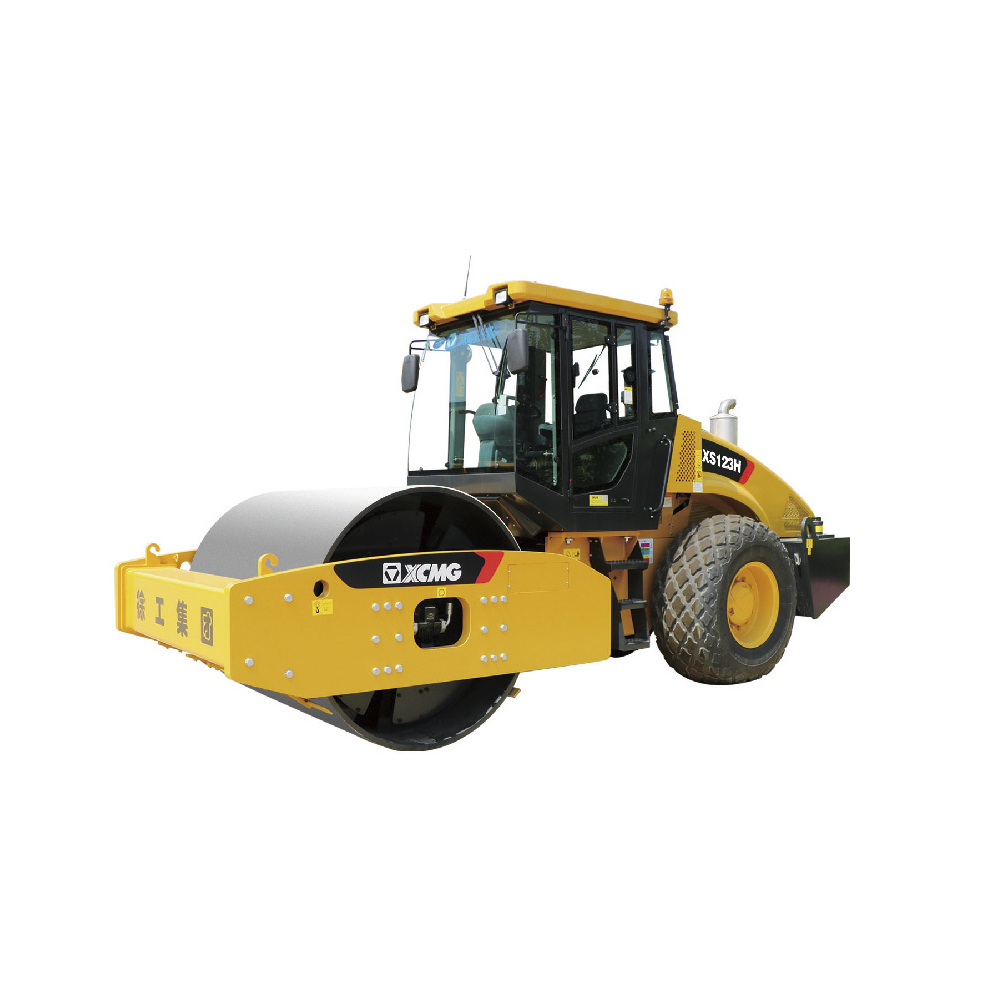The image features a prominent yellow steamroller positioned against a stark white backdrop, occupying almost the entire frame. Key details include a large gray roller at the front, flanked by yellow brackets. On these brackets, a black sticker with the letters "XCMG" in white font is visible. This branding is also seen on a black background with a red accent on the side of the vehicle. The steamroller model, partially obscured but identifiable as "XS123H", is indicated near the rear. The steamroller's cabin, situated above and to the right of the roller, features a yellow roof with a black frame and large windows on all sides, offering visibility for the driver. This cabin area includes two rear-view mirrors. The vehicle also has black tires with yellow hubcaps, a silver smokestack, and an access ladder leading to the cab. The steamroller's color palette comprises yellow, black, gray, silver, and small hints of white and red. Additionally, the presence of possibly Asian script suggests its origin, emphasizing its functional and industrial design.